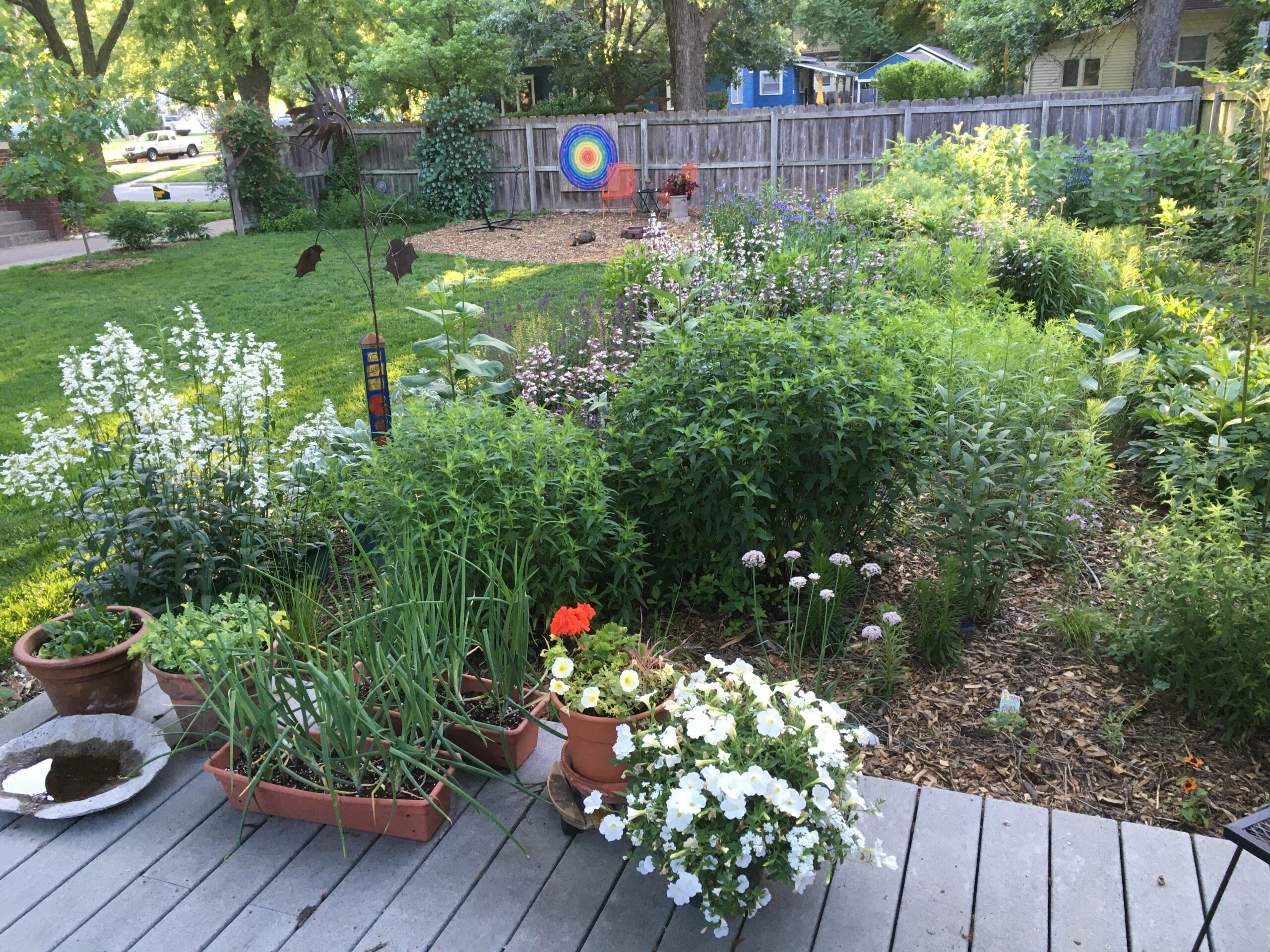The photograph captures a vibrant and meticulously maintained outdoor garden bathed in bright sunlight. The garden features an array of lush greenery and colorful blooms, showcasing the thriving life of late spring or early summer. Positioned on a grayish wooden deck are a variety of potted plants, some in traditional clay pots and others in rectangular trays. Among these, some plants appear to be vegetables, possibly onions, while others boast vivid flowers.

Adjacent to the deck is a larger garden brimming with diverse plants and flowers. The floral display includes an assortment of white blooms, small purple-topped flowers, and several green bushes adorned with white accents. A backdrop of little yellow flowers is interspersed with splashes of pink and purple, creating a lively and colorful scene. The ground between the plants is meticulously mulched, devoid of weeds, indicating a well-tended space where every plant has been intentionally placed.

The garden extends all the way back to a wooden fence, beyond which more bushes can be seen. This fence is decorated with a colorful target-like ornament featuring concentric circles in red, yellow, blue, and purple hues. Near this vibrant decoration lies a small rock garden with a sparse selection of plants.

In the lower right corner of the image, the edge of a chair hints at a cozy seating area for enjoying the picturesque view. The front of the garden opens towards the street, where parked cars and a sidewalk bordered by a neatly kept grassy lawn are visible in the distance. All these elements come together to present a healthy and dynamic garden, a testament to the gardener's dedication and care.